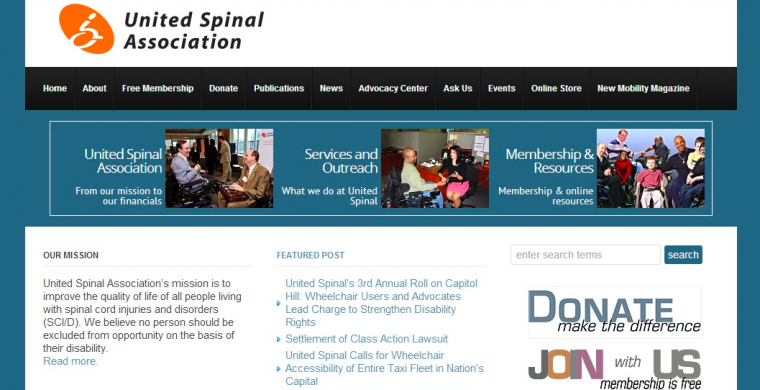The image showcases a webpage displayed on a laptop, specifically from the United Spinal Association. At the very top of the webpage, there is a banner featuring a white background with black text. The banner also incorporates the United Spinal Association's logo in orange. Just below this banner is another, with a black background and white text, serving as the main navigation menu. The menu options are: "Home," "About," "Free Membership," "Donate," "Publications," "News," "Advocacy Center," "Ask Us," "Events," "Online Store," and "New Mobility Magazine," which users can click on to explore different sections of the website.

Proceeding down the page, there are several photographs depicting individuals involved with the association along with various clickable elements that provide more information. Further down, there is a section with text on a white background that includes details on donating and how to become a member of the United Spinal Association. The overall layout is well-organized and visually appealing, facilitating easy navigation and access to important information.